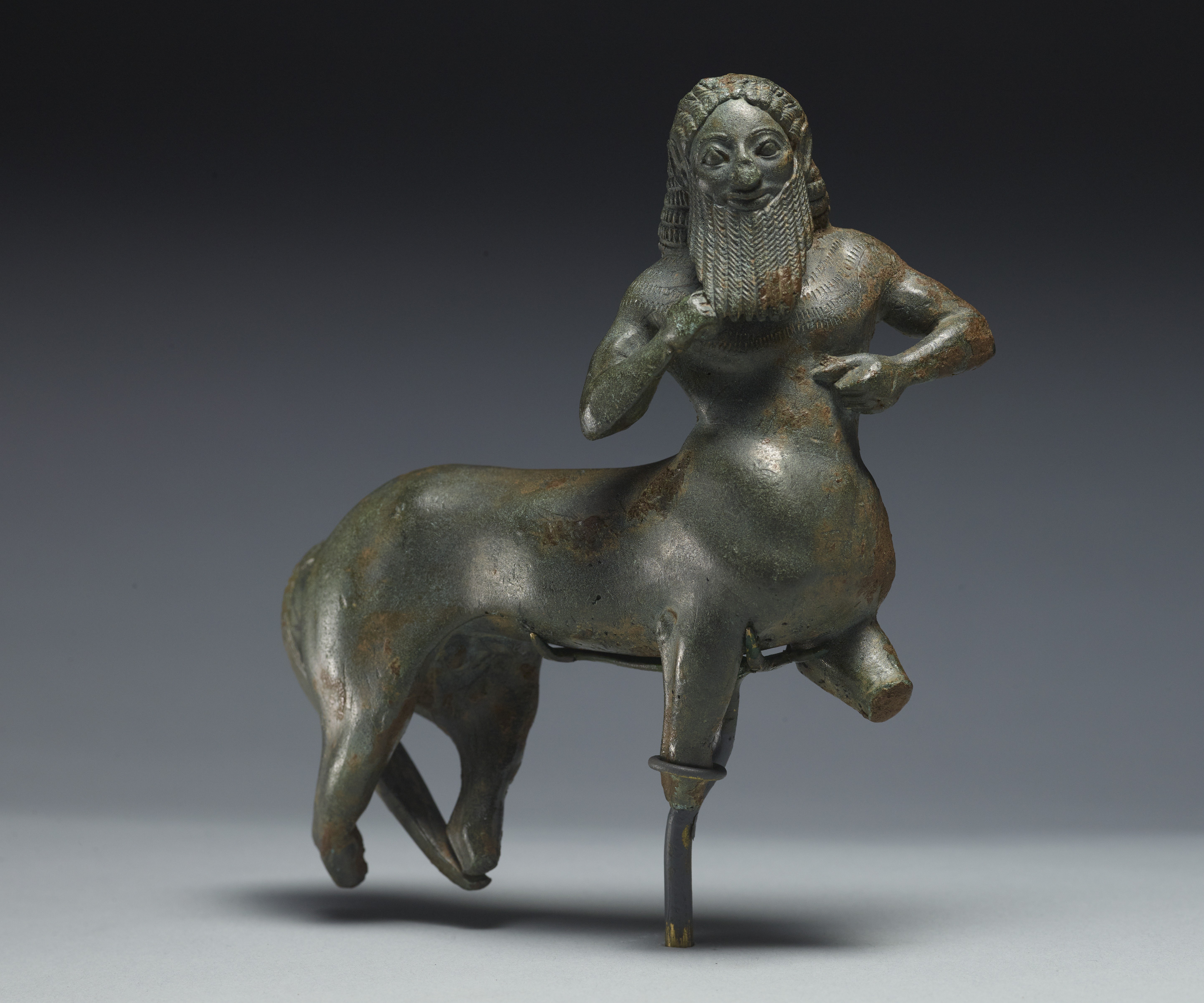This horizontal rectangular image features a detailed metal sculpture of a centaur, expertly placed on a pristine white surface against a gray background. The centaur's hindquarters, resembling a horse, merge seamlessly with the upper body and head of a man. Notably, the man has a long beard and either long braided hair or perhaps a hat. His face, adorned with glasses and a broad smile, exudes joy. Muscular and strong, the centaur is missing one of its front legs, instead having a peg leg, while the other leg is cut off into a stump, adding a layer of intrigue and character to the piece. The metal of the sculpture is a dark, slightly rusted silverish hue, giving it an ancient, timeless feel—almost as if it originated from the era of ancient Greece. The gray background transitions from black at the top to white at the bottom, enhancing the sculpture’s striking presence.